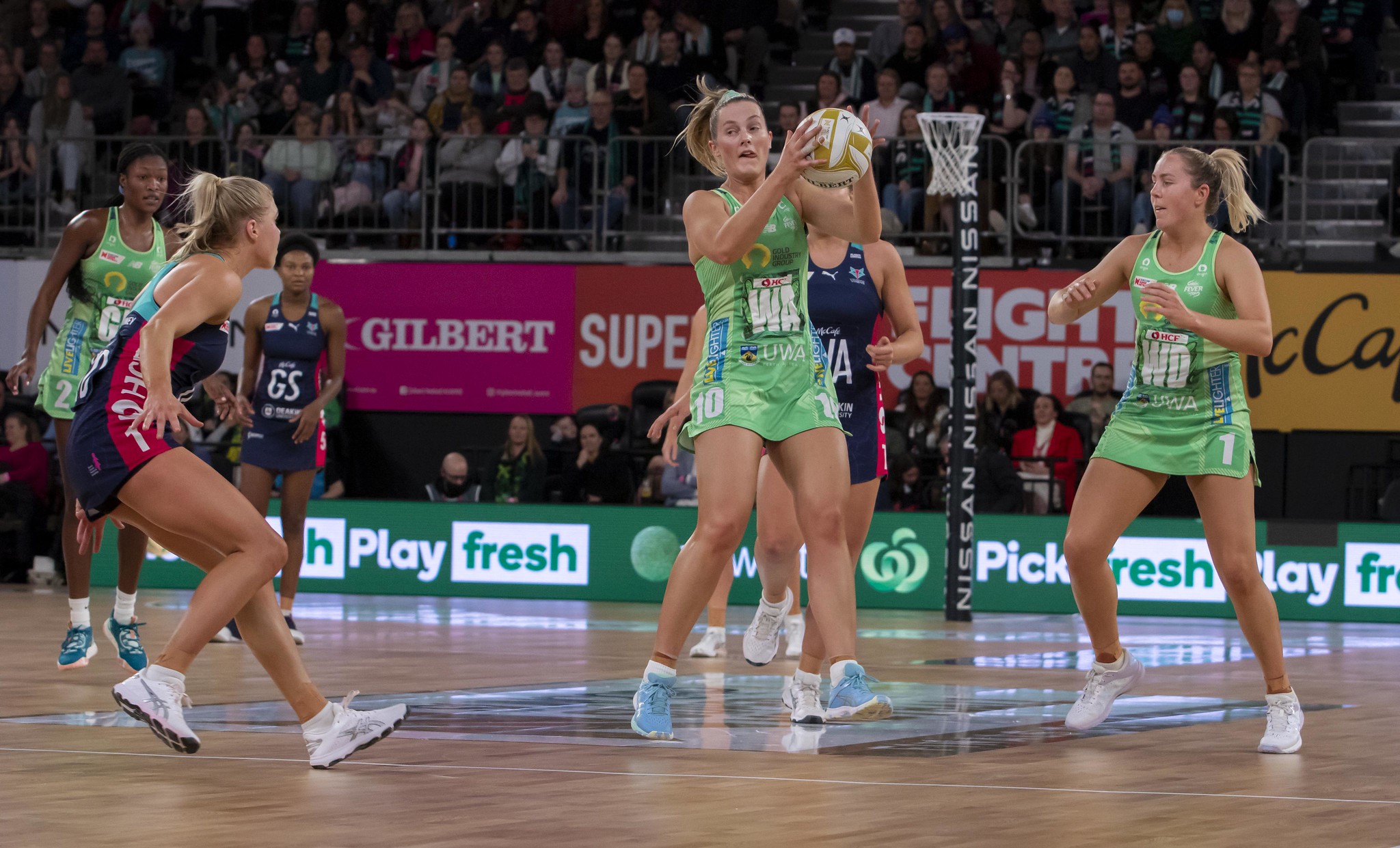The image captures an intense moment during a volleyball game, with a hardwood floor underfoot and a vibrant atmosphere in the background. A woman, donning a green jersey emblazoned with "WA" and the number 10, stands at the center of the action. She is captured mid-motion, holding a yellow and white volleyball, her mouth open as if calling out. Around her are two teammates in matching green jerseys and three opponents in blue uniforms with red accents rushing towards her, all engaged in the fast-paced dynamics of the game. The scene is set against a backdrop of lively spectators, with photographers, reporters, and additional onlookers situated on the sidelines. Banners advertising brands like Gilbert, McCafe, and Super are visible across the bleachers, adding to the energetic ambiance. The setting includes a singular hoop on a pole at the back, marked with "Nissan," indicating a multi-purpose sports environment.